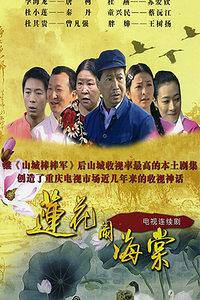The poster, likely from one of the Asian nations such as China or Korea, features a prominent yellow background with Asian text that could be Chinese or Korean. At the center, there are six individuals – three men and three women – arranged in a V formation. The leading figure, a man wearing a blue coat and a blue ball cap, stands in front of the others who appear to be of varying ages and possibly different occupations. The upper part of the poster showcases a silhouette of birds flying in the sky, adding to the visual appeal. Below, vibrant watercolor flowers grace the design, including a prominent pink flower on the center left and several grey-toned flowers along the bottom. The poster, which possesses a somewhat faded and older appearance, also incorporates additional Asian text in black, red, and bright yellow hues.